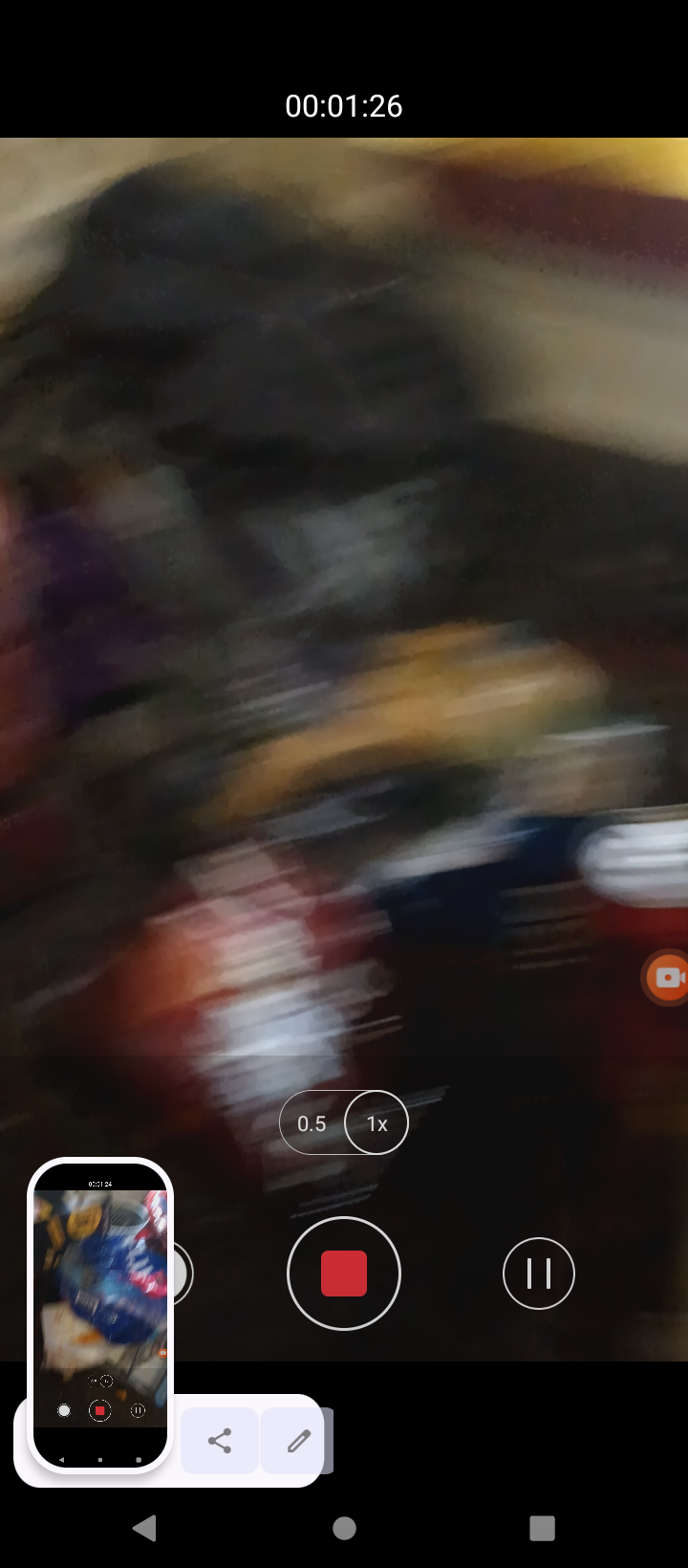A screenshot captured from a smartphone video recording, showing the camera app interface at the 1 minute 26 second mark (00:01:26) on a black rectangular background akin to a smartphone screen. The main screen, extremely blurry and unrecognizable, displays an array of moving colors, including yellow, red, blue, green, white, purple, and gray. The red record button occupies a central position at the bottom, flanked by magnification options (0.5x and 1x) and a pause button to the right. A picture-in-picture inset at the lower left replicates the blurred main image, indicating a potential FaceTime call or screen recording with identical hues: black, yellow, red, blue, and white. The icon for sharing or editing this content appears at the bottom, affirming it is a screenshot taken from the phone's active recording function.